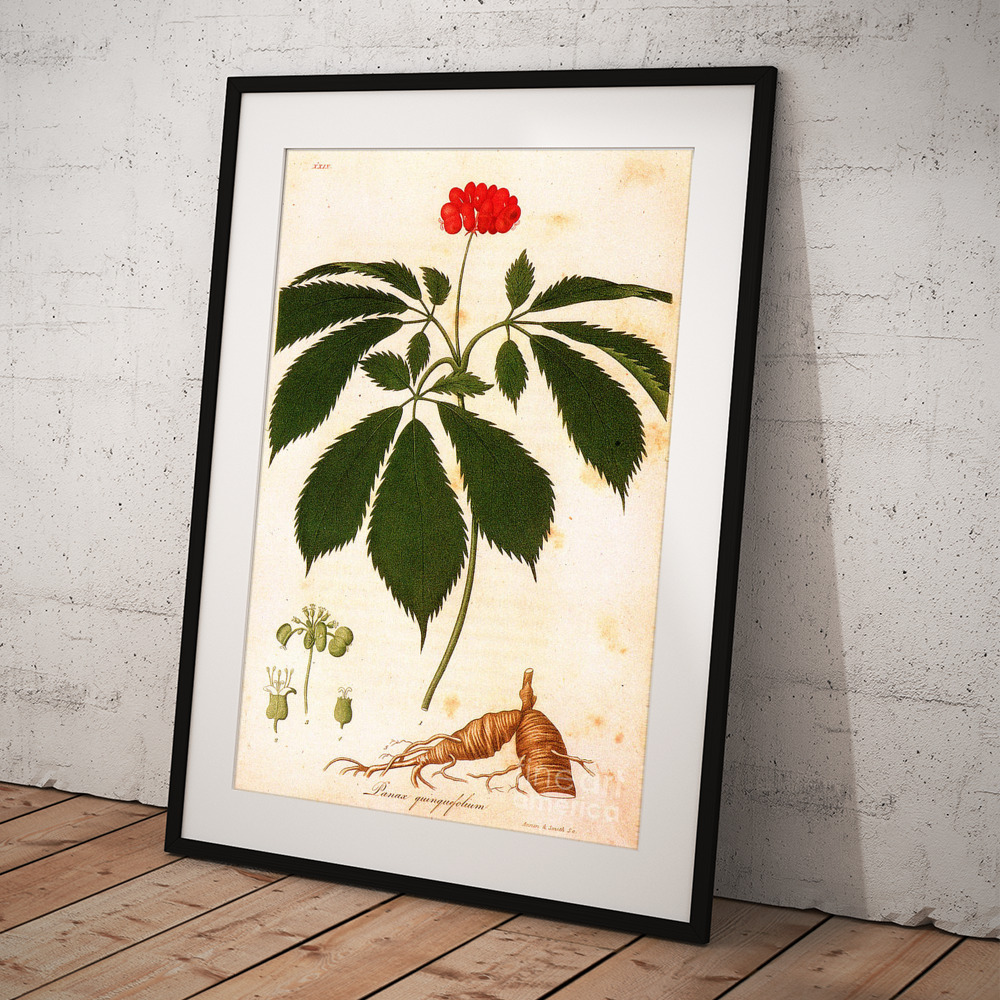A large, framed botanical illustration leans against a whitewashed stone wall on a blonde wood floor. The black frame encompasses a white matting that surrounds a detailed, classic drawing of a flowering plant on a vellum-like background. Central to the illustration is a robust stem adorned with jagged-edged leaves and a prominent red flower, possibly a geranium. The root system of the plant, depicted in the bottom right, shows extensive offshoots that suggest how the plant establishes itself in the soil. The bottom left features a close-up of the floral structure, likely illustrating the development from a budding stage to a fully blossomed flower. Despite some unreadable text and a watermark on the image, the illustration's intricate details and dated style convey a sense of historical botanical artistry.